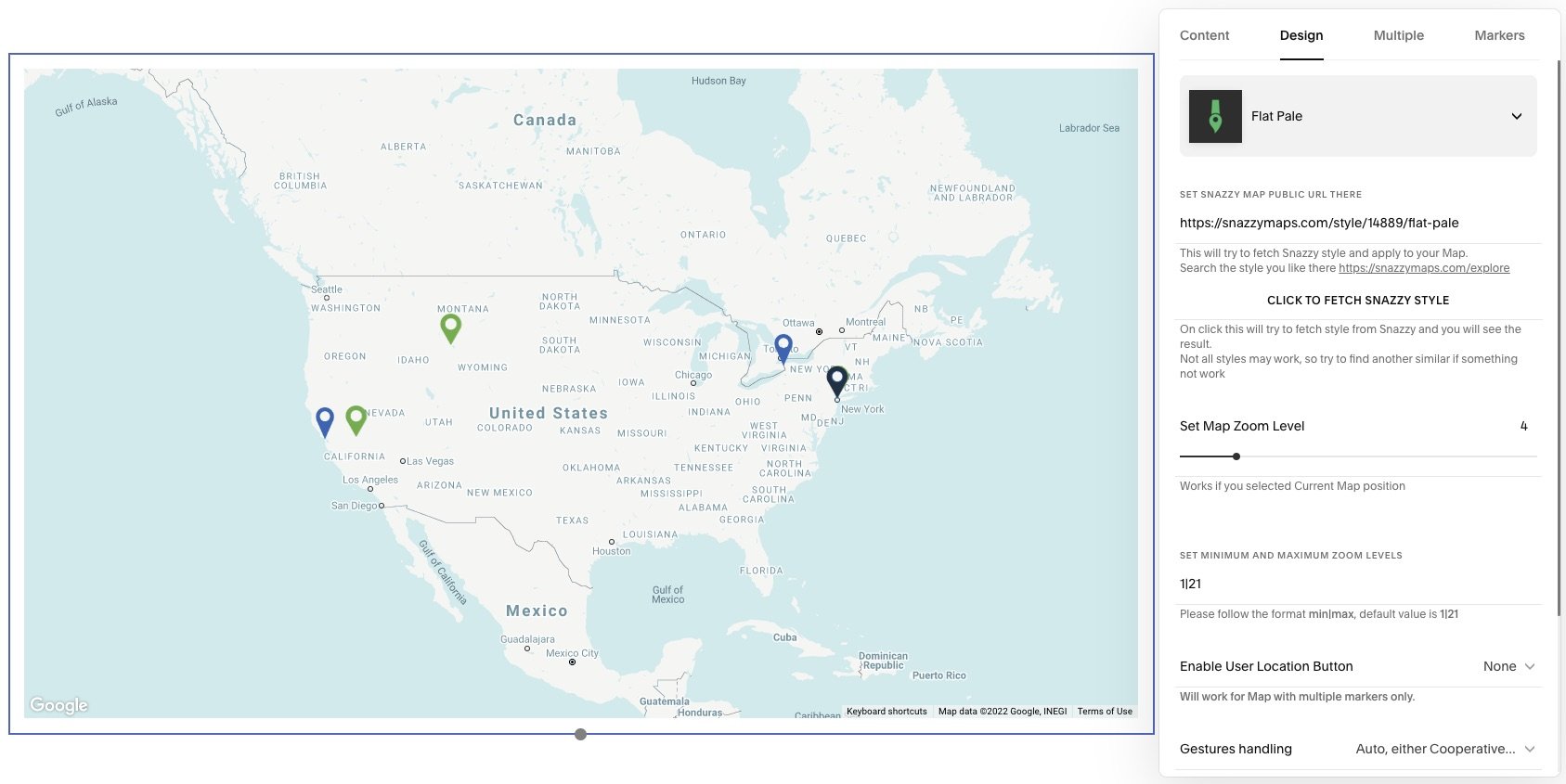Screenshot of a digital map featuring the United States, Canada, and Mexico on a white background. The map is adorned with five location icons: two in green, two in blue, and one in dark blue, each representing different points of interest. The map also includes labels for 'Content', 'Design', 'Multiple', and 'Markers', alongside several pieces of information. A black hyperlink is visibly embedded within the map's interface. Dynamic elements like 'Click to Fetch' are incorporated with a stylish flair. Additional details include references such as 'Saturday', 'SAT', 'Map Zoom Level', and options to 'Set Map Zoom Level'. A shaded bar, possibly indicating a loading or progress metric, is displayed, filled to approximately 15-20% capacity.